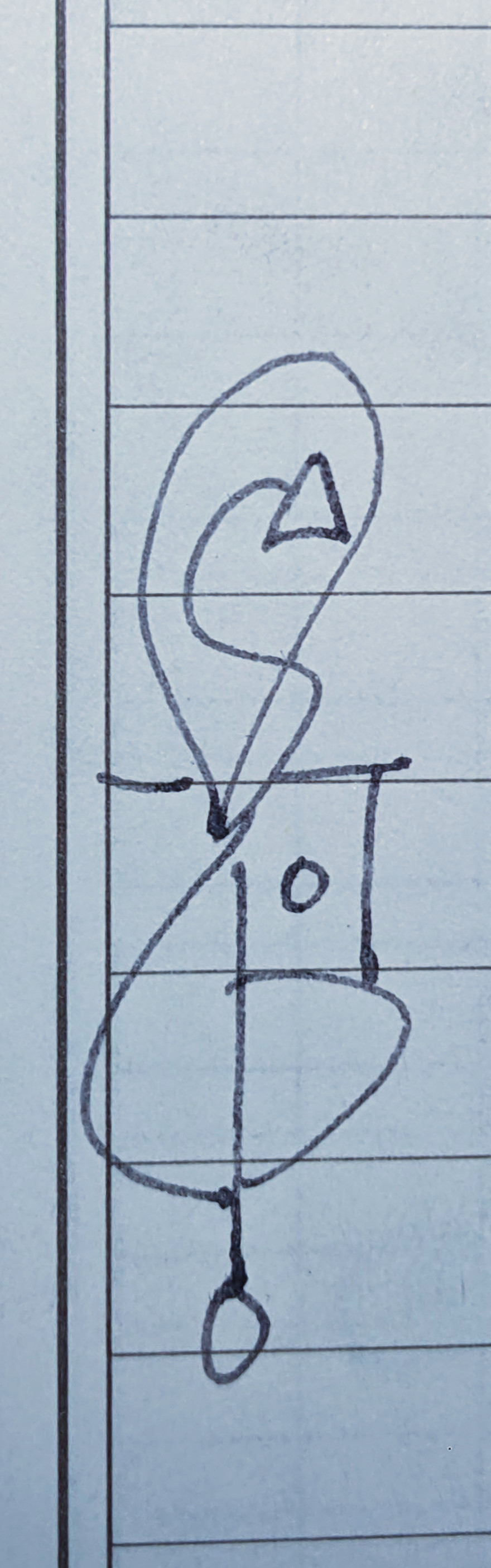This is an image of a hand-drawn sketch rendered in somewhat faded black ink on a sheet of lined paper. The paper exhibits approximately 10 evenly spaced horizontal lines, along with faint vertical guidelines. The drawing prominently features an arrow pointing to the right, indicating some form of directional emphasis. Additionally, the composition includes numerous areas of scribbling, adding a textured, chaotic element to the artwork.

Central to the drawing is a small circle situated roughly at the midpoint of the page. Adjacent to this, there is a T-shaped figure, its horizontal component aligning parallel to the paper’s lines. At the bottom of the sketch, a significantly larger circle is meticulously outlined. This larger circle is connected to the primary drawing by a vertical line over an inch in length, suggesting a form of linkage or connection between the elements.